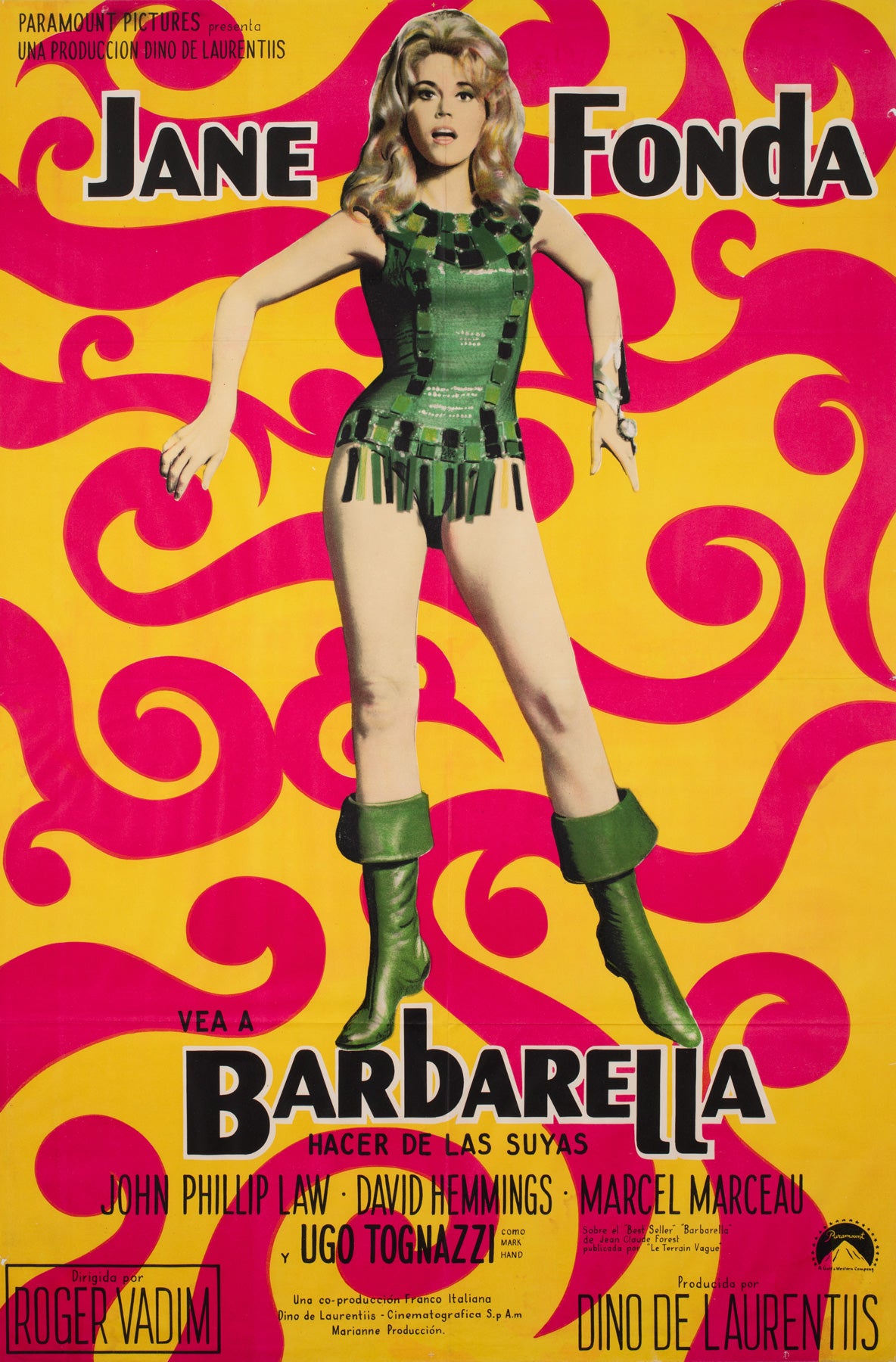This is a vintage poster of the 1960s movie "Barbarella." The background of the poster is yellow adorned with pink, red, and purple psychedelic scroll patterns. In the center stands a striking image of Jane Fonda. She is portrayed in a short, green mini dress with frills at the bottom, paired with matching green cuffed boots. Fonda's blonde hair is styled in a bouffant, and she wears jewelry on her left arm. Her pose is dynamic, with arms extended to her sides and her legs in a pointed toe-tip stance, conveying a sense of action and surprise as she looks directly at the viewer.

The top of the poster features Jane Fonda's name in bold black lettering. Beneath her feet is the title "Barbarella," along with additional text listing some of her co-stars: John Philip Law, David Hemmings, Marcel Marceau, and Ugo Tognazzi. The production credits include the prominent names of Dino De Laurentiis and Roger Vadim. The bottom of the poster displays the phrase "Vea Barbarella" and includes the Paramount logo, indicating the studio behind the movie. This colorful and detailed poster perfectly captures the essence of the sci-fi classic and its era.